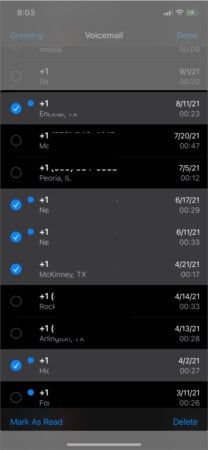This image captures a smartphone screenshot featuring a voicemail interface against a black background. At the top left, the time is displayed as "8:03" in white text. On the top right, standard smartphone indicators such as signal bars, a Wi-Fi signal, and a low battery icon are visible.

The central area, slightly grayed out, is titled "Voicemail." The first voicemail entry shows a minimal detail with a "+" sign adjacent to the numeral "1." To the right, it shows the date "9/1/21." The next voicemail entry has a blue circle with a checkmark, indicating it has been heard or marked. This entry lists "+1" and more detail about the voicemail: "8/11/21" for a duration of "23 seconds."

Following this, there are two unselected voicemail entries:
1. "+1" with the date "7/20/21" for "47 seconds."
2. "+1" with the date "7/5/21" for "12 seconds."

Beneath these, three selected voicemails marked with blue circles and white checkmarks appear, all labeled "+1." The dates and durations of these voicemails are:
1. "6/17/21" for "29 seconds."
2. "6/11/21" for "33 seconds."
3. "6/21/21" for "17 seconds."

Further down, the list contains two more unchecked voicemail entries:
1. "4/14/21" for "33 seconds."
2. "4/13/21" for "28 seconds."

Next is a selected voicemail, as indicated by the blue circle with a checkmark:
- "4/2/21" for "27 seconds."

Finally, at the bottom, there is an unselected voicemail labeled:
- "3/11/21" for "26 seconds."

The interface concludes with options in blue text: "Mark as read" and "Delete."